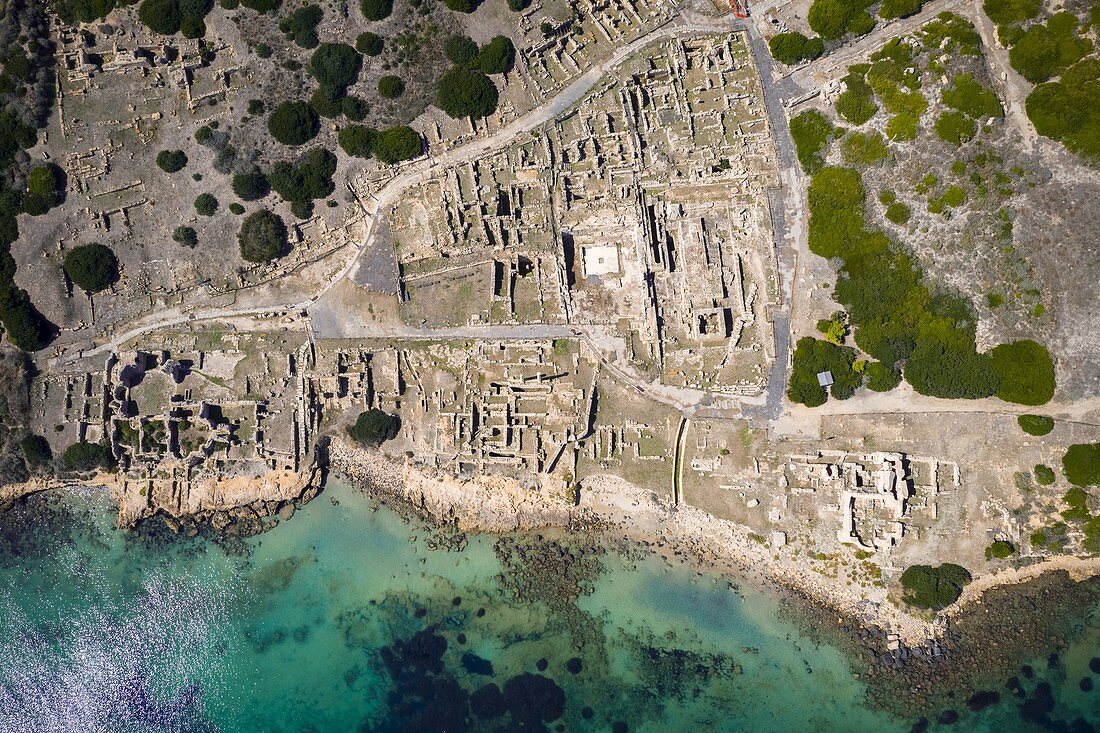The image is an expansive aerial photograph capturing the remnants of an ancient coastal city, likely taken from a significant height using a drone or helicopter. The central focus is the sprawling ruins marked by numerous rectangular and incomplete walls, hinting at a historical site rich with archaeological significance. These ruins are predominantly gray, contrasting with the lush green bushes and trees scattered along the perimeter. The lower part of the frame reveals clear blue coastal waters, reminding us of the city's once strategic and bustling nature. The overall scene, viewed from a high vantage point, emphasizes the vast scale of the ancient city and provides a detailed glimpse into its past grandeur amidst its now-decayed state.